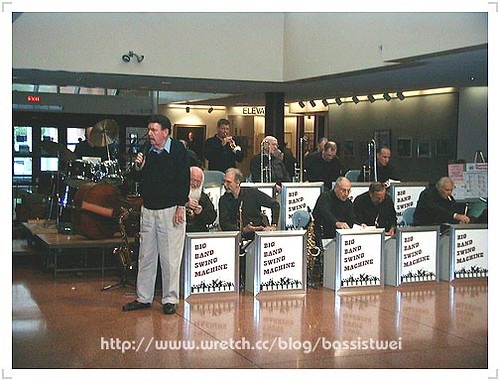The photo captures an indoor setting featuring a live performance by a large band called the "Big Band Swing Machine." On the left, a man is speaking into a microphone, dressed in gray pants and a black shirt over a blue undershirt. Surrounding him is a group of around 10 to 12 band members, each positioned behind individual podiums adorned with banners that read "Big Band Swing Machine." The front row consists of five men, including the third member from the left who has a saxophone beside him. The back row has additional musicians, most of whom are holding or seated near trumpets. Behind the speaker, there's a drum set and a large cello or double bass. A URL at the bottom of the image reads "www.reg.cc.com/blog/bassistTWEI," suggesting further information about the band can be found online. The overall scene hints at a vintage concert setting with a well-organized ensemble ready to perform.